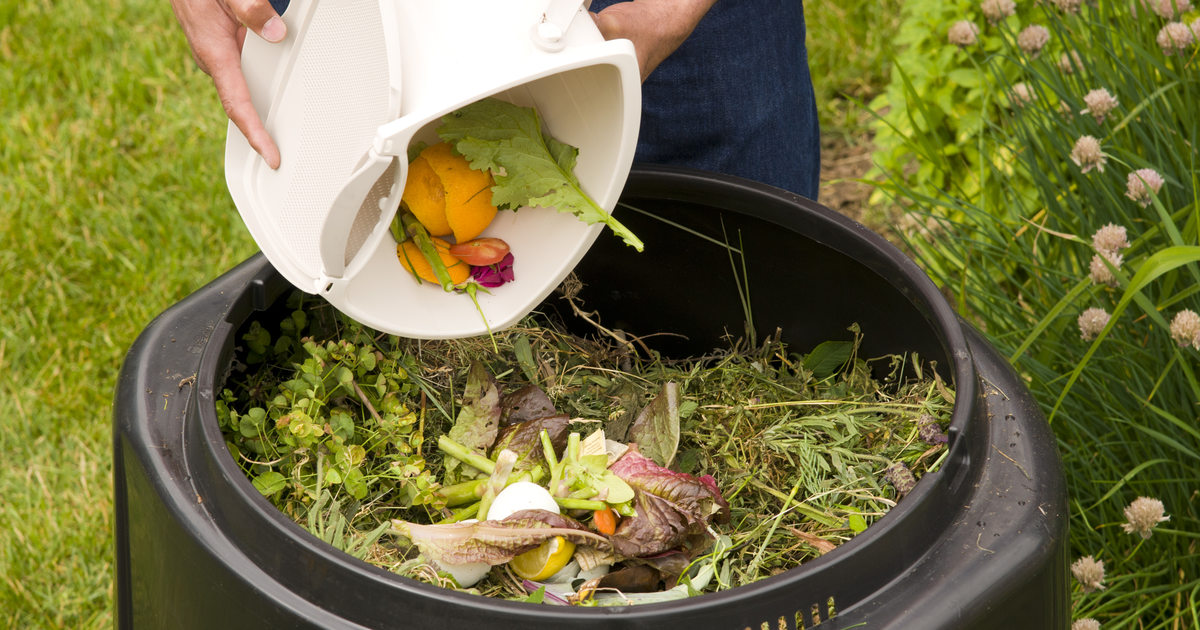This photograph captures a composting operation in a green, landscaped area, likely a backyard. Central to the image is a large, round, black plastic barrel filled with compostable debris, including grass clippings, rotten cabbage pieces, orange and carrot peels, lettuce, lemon pieces, and a tomato slice. The black barrel serves as a receptacle for organic waste. To the left, a vibrant green lawn adds to the lush setting, while the right side features tall grass and pinkish-white flowers resembling clovers. A person, only visible by their hands clad in blue denim, is seen holding a white bucket and pouring the compostable materials into the barrel, indicating active participation in composting. This scene, bathed in the warm light of spring or summer, clearly illustrates a home composting setup.